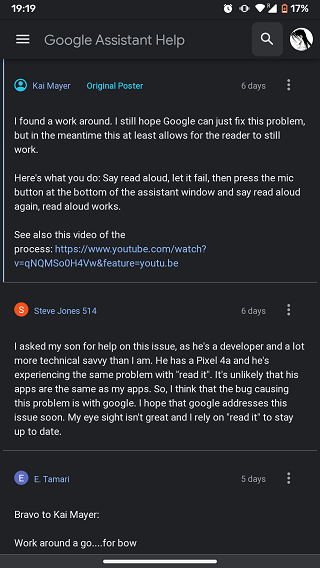Screenshot of a Google Assistant Help Forum captured on a mobile device at 19:19 with a battery level of 17%. The forum thread is initiated by Kai Meyer who shares a temporary solution for an issue with the "Read Aloud" feature. Kai's post reads: "I found a workaround. I still hope Google can just fix this problem, but in the meantime, this at least allows for the reader to still work. Here's what you do. Say 'Read Aloud,' let it fail, then press the mic button at the bottom of the Assistant window and say 'Read Aloud' again. 'Read Aloud' works. See also this video of the process," followed by a YouTube video link.

Beneath Kai's post, user Steve Jones 514 comments: "I asked my son for help on this issue, as he's a developer and a lot more technically savvy than I am. He has a Pixel 4a, and he's experiencing the same problem with 'Read It.' It's unlikely that his apps are the same as my apps, so I think that the bug causing this problem is with Google. I hope that Google addresses this issue soon. My eyesight isn't great, and I rely on 'Read It' to stay up to date."

Another user, E. Tamari, adds a response 5 days ago: "Bravo to Kai Meier. Workaround a go... for Beau."

The entire thread is displayed in white text on a black background.